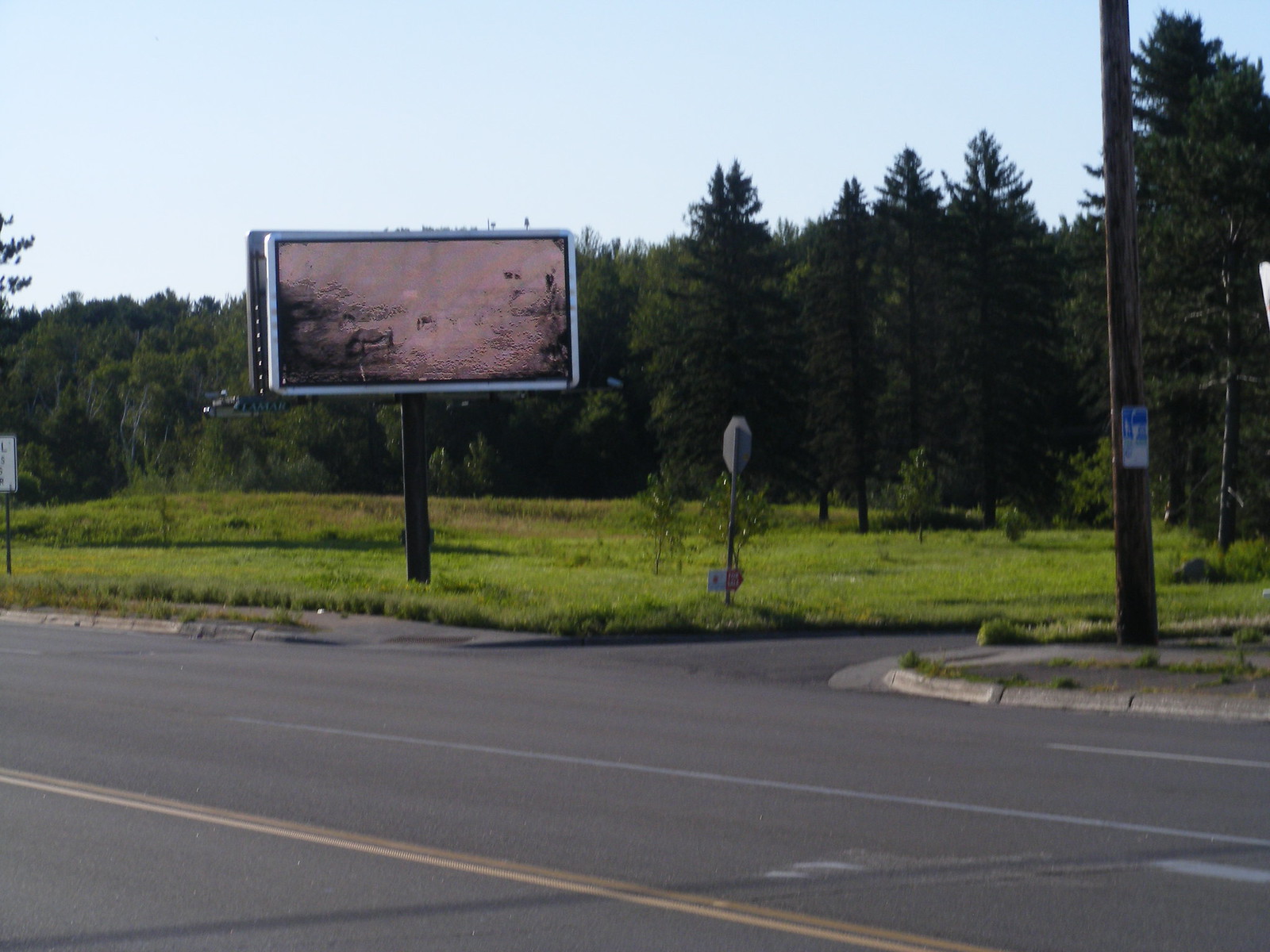The image depicts a deserted road with a weathered, blank roadside sign standing to the right side of the blacktop surface. The road, marked by two solid yellow lines down the center and a long white line on the right, leads to a small intersection featuring a stop sign. No vehicles are present, enhancing the sense of solitude in this scene. In the background, dense foliage and tall pine trees create a lush, forested backdrop, with wild grass growing thickly around the base of the ancient, faded sign. This tranquil setting in nature evokes a sense of timelessness and quietude.